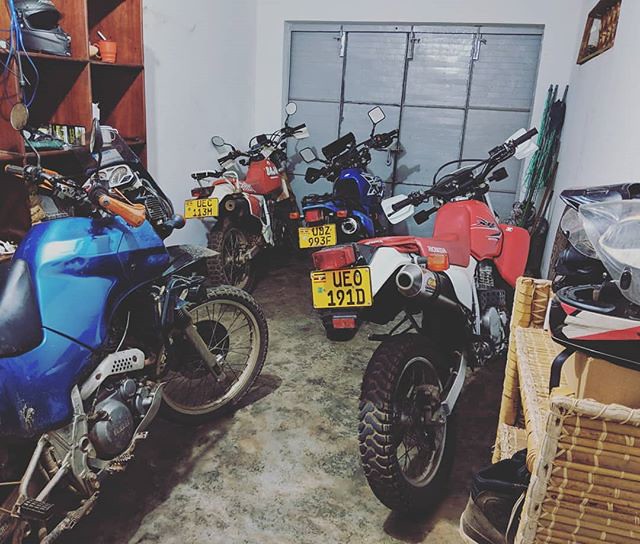This photograph captures the detailed interior of a garage, featuring a range of storage items and several motorbikes. The garage floor is covered in a granite-like surface with a mixture of black, white, gray, and tan. There are four motorbikes present, each with yellow license plates and leaning to the left. The motorbike on the far left is blue, followed next by a red and white one. In the foreground on the right, there is another red and white bike, and beside it is another blue bike. The motorbikes' license plates include UE01910, UE2993F, 2284, among others.

The walls of the garage are white, and the metal garage door is grey. On the left side of the image, there is a set of dark brown wooden shelves stacked with various items, including a black motorcycle helmet. To the right, there is a light brown wicker shelf holding more helmets—one black and another black, white, and red—as well as a pair of brown and black shoes on the bottom shelf. Higher up on the wall to the right is a brown plaque with white details. Additionally, there seems to be a panelled window with shutters behind the bikes, and some green folding chairs visible on the right side along with what could be a picture frame. The overall ambiance of the garage suggests a well-organized space dedicated to motorbike storage and maintenance.